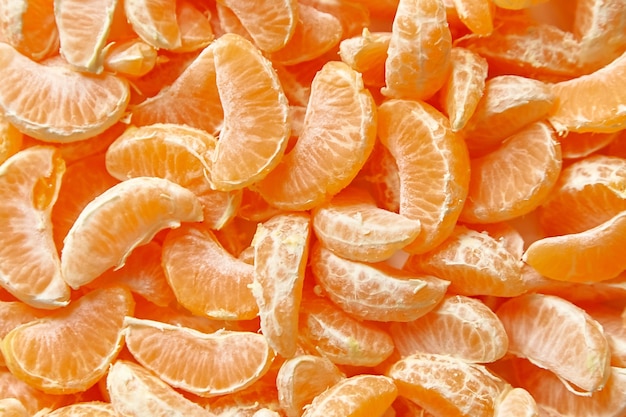This color photograph is a close-up image featuring numerous segments of mandarin oranges, creating an overwhelmingly bright and vibrant orange display. The segments appear to be piled haphazardly into a confined space, indicating they may have been dumped into a bin or a bucket. The image showcases around two dozen or more juicy mandarin segments, each in various positions and orientation, some with visible white stringy pith sticking out. The segments range from light to dark orange, contributing to the vivid color palette. There are no visible humans, animals, structures, or machines in the photo, focusing solely on the mandarin slices, which appear fresh and appetizing.